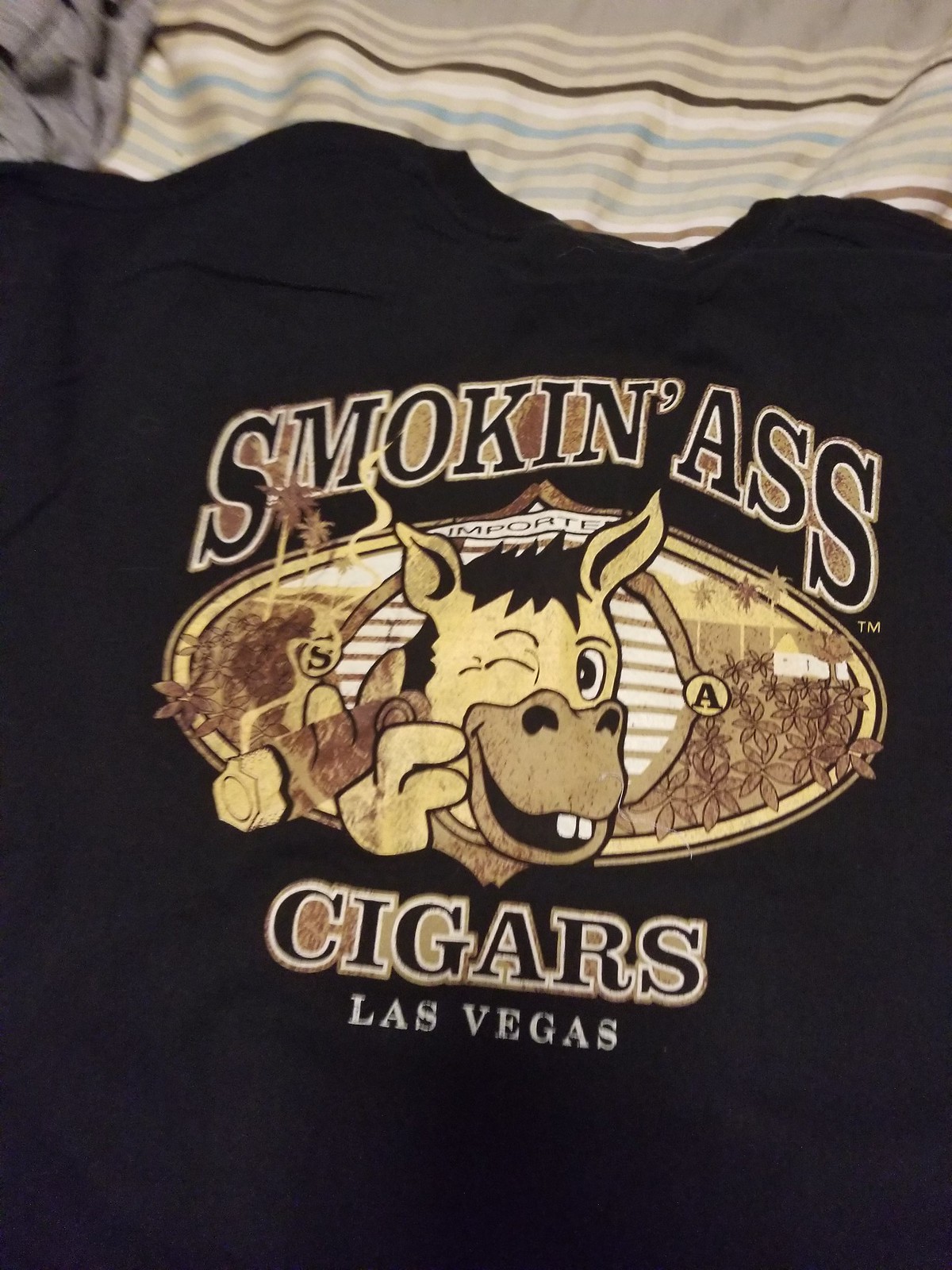The image showcases a black t-shirt resting on a surface resembling a bed. The shirt prominently features the text "Smoking Ass" in a brown sepia font. Below the text is a playful illustration of a donkey, which is winking with its right eye and smiling, revealing its two front teeth. The donkey is depicted holding a cigar with its right hoof. Encircling the cigar, the words "Cigars" and "Las Vegas" are also displayed in the same brown sepia font. The overall aesthetic of the design combines humor and a vintage feel.